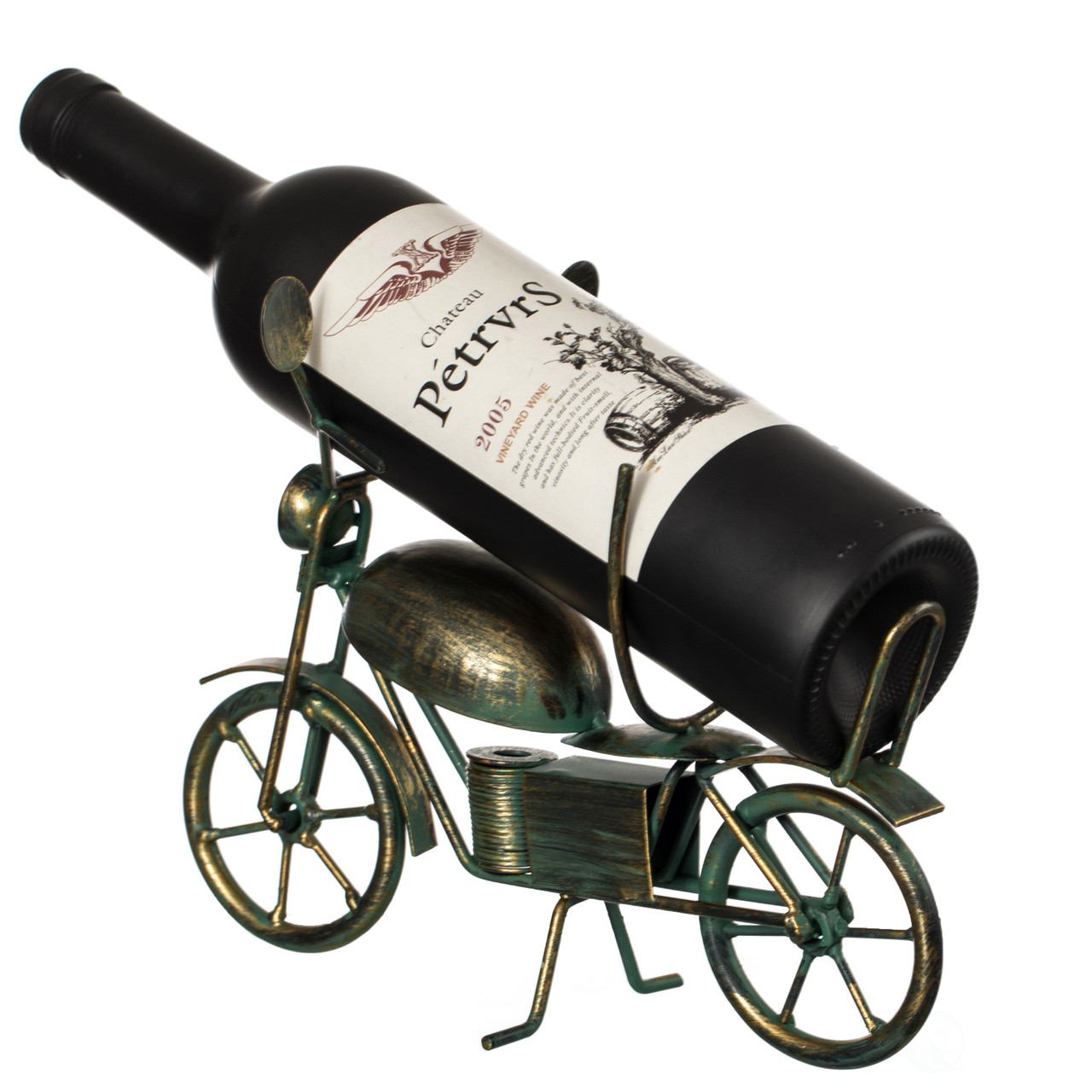This product image features a uniquely designed wine holder styled as a vintage bicycle or motorcycle, meticulously placed against a pure white background that has been edited to remove any distractions. The holder itself is a striking piece, primarily bronze with brushed accents of greenish gold and turquoise, giving it a slightly rustic appearance with an artistic flair. The bicycle stand, complete with two wheels, holding arms instead of a seat, and its own supportive stand, securely cradles a classic black wine bottle. The bottle, a 2005 Chateau Petreu wine, showcases a white label adorned with intricate designs, including a dark reddish symbol at the top, a central black tree flanked by an oak barrel, and elegant script denoting the wine’s prestigious vineyard origin.